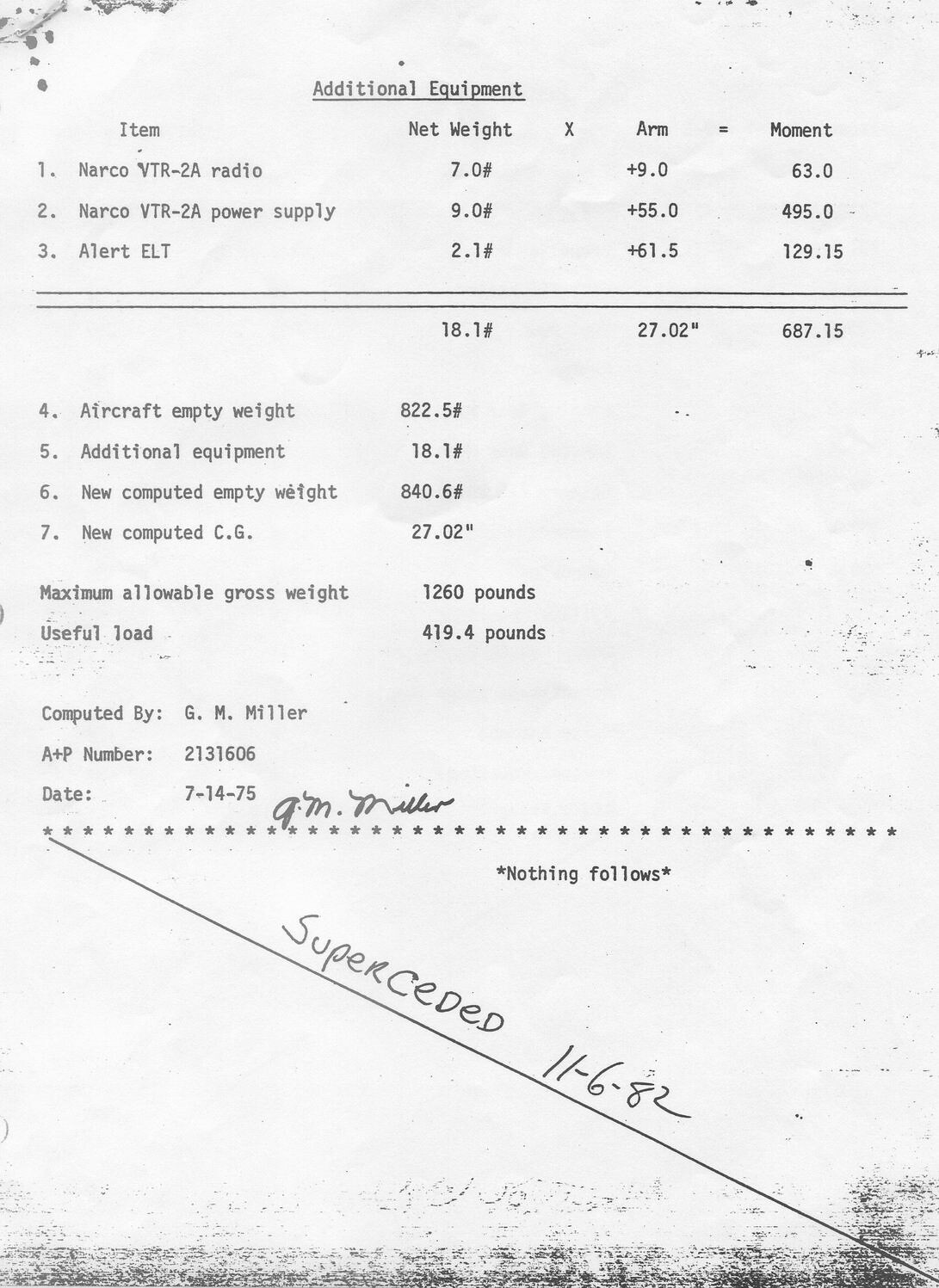The image depicts a scanned or photocopied receipt on a white background, with a clear heading at the top, underlined, reading "Additional Equipment." The receipt is formatted with columns labeled "Item," "Net Weight," "Arm," and "Moment," and items listed down the side numbered 1 to 3 in the first section. 

1. **Number 1:** Narco VTR2A Radio; Net Weight: 7.0; Arm: +9.0 (in 60 units); Moment: 63
2. **Number 2:** Narco VTR2A Power Supply; Net Weight: 9.0; Arm: +55.0; Moment: 495
3. **Number 3:** Alert ELT; Net Weight: 2.1; Arm: +61.5; Moment: 129.15

Below these entries, a second section continues with:

4. **Number 4:** Aircraft Empty Weight; Net Weight: 822.5
5. **Number 5:** Additional Equipment; Net Weight: 18.1
6. **Number 6:** New Computed Empty Weight; Net Weight: 84.6
7. **Number 7:** New Computed C.G.; Arm: 27.02

Following this, it states:

- **Maximum Allowable Gross Weight:** 1,260 pounds
- **Useful Load:** 419.4 pounds

The receipt is signed off with "Computed by G.M. Miller," followed by "A&P Number: 2131603," and "Date: 7-14-75." There's a signature next to the date, attributed to G.M. Miller. At the bottom, a starred line leads to the note "Nothing Follows." Handwriting over the receipt indicates it was "Superseded 11-6-82."